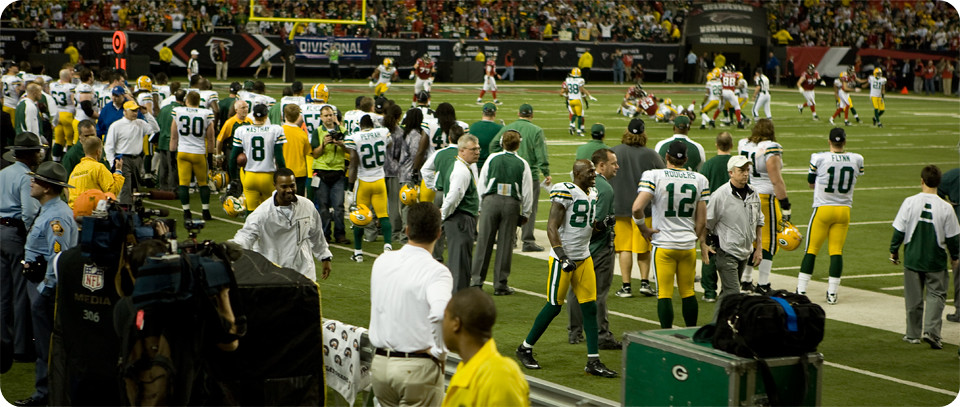The image captures a vibrant moment on the sideline of a Green Bay Packers football game. The perspective is from behind the bench, looking up towards the left. Dominating the foreground are Packers players in their iconic white jerseys with green numbers and yellow pants, including notable numbers such as 12 (Aaron Rodgers), 10, and 80, all walking to the right. The sideline is bustling with activity; coaches dressed in gray slacks and green and white shirts, along with medical and football equipment, including a green equipment box marked with a 'G,' a black bag on top of it, and towels on the bench, are visibly spread around.

Off to the left side, there are a few policemen keeping an eye on the crowd, which stretches into the background, filled with enthusiastic fans cheering from the stands. The photo also captures the distinct yellow goalposts in the upper left corner of the frame. On the field, the action unfolds with both the Green Bay Packers and their opponents, the Atlanta Falcons, engaged in a play. The Falcons players, identifiable by their red jerseys and black helmets, include numbers 88 and 83, are in the midst of the game, with several players on the ground.

Overall, the scene is a dense tapestry of game-day elements: players, coaching staff, equipment, and a lively crowd all focused on the unfolding football action in a stadium that’s teaming with energy.